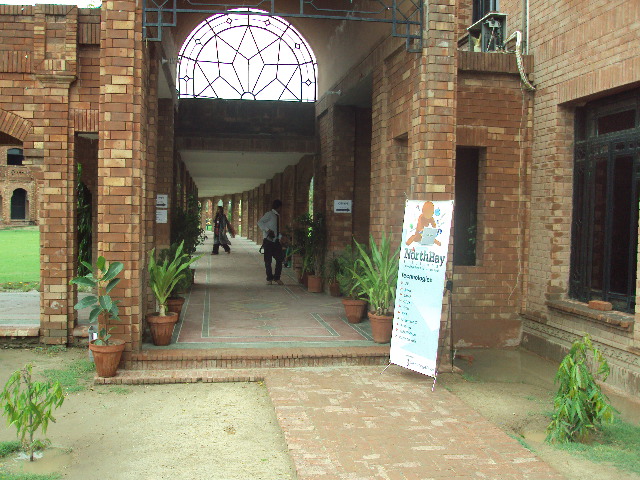This image depicts the entrance to an outdoor hallway of an old, historical-looking school building made of brown stone. The long hallway features stone arches and a beautifully crafted concrete pathway in shades of grey, red, and yellow bricks. Potted plants are placed near every column on both sides of the hallway, adding a touch of greenery. Flanking the entranceway, two sturdy columns rise and frame a semi-circular stained glass arch with intricate triangle and star patterns, bathed in sunlight. Above the entrance is a black wrought iron feature and a prominent white sign reading "North Bay Technologies." In front of the hallway, two trees stand tall, contributing to the serene atmosphere. Two students can be seen walking through the shaded corridor, adding life to the stillness of the scene.